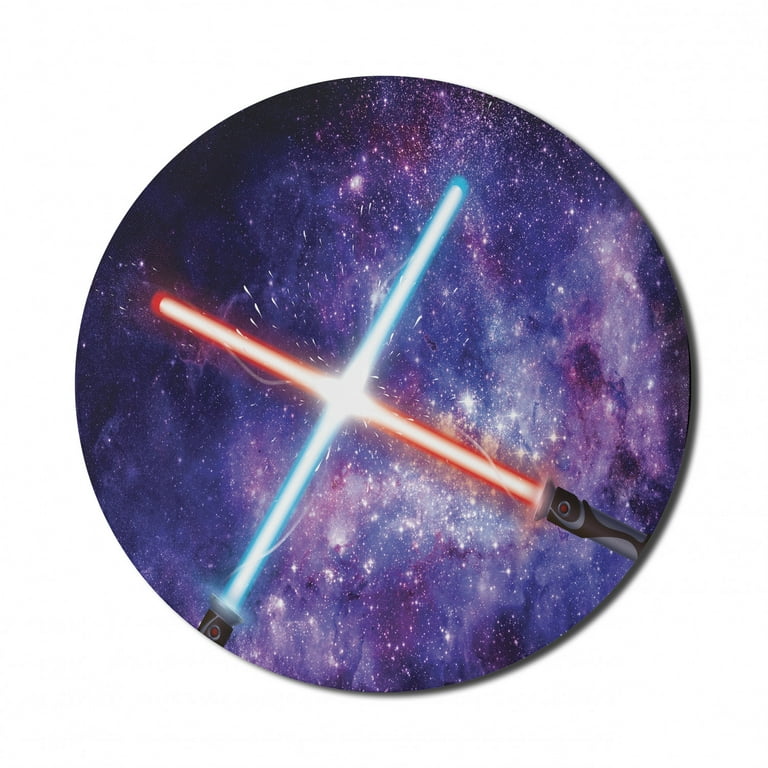This image is a perfect circle, resembling a round pin or possible art piece, with a subtle shadow beneath it. The background is a stunning interstellar scene, featuring a rich tapestry of colors, including deep blues, purples, and black, interspersed with bright white spots resembling stars. Dominating the center, two detailed lightsabers—one blue and one red—cross each other in an X formation, as if engaged in a fight. The point where they intersect glows with intense white light, emphasizing the clash. The lightsabers' handles are gray and black, adorned with small red buttons, which likely serve as activation switches. This image beautifully merges cosmic and iconic elements into a visually striking design.